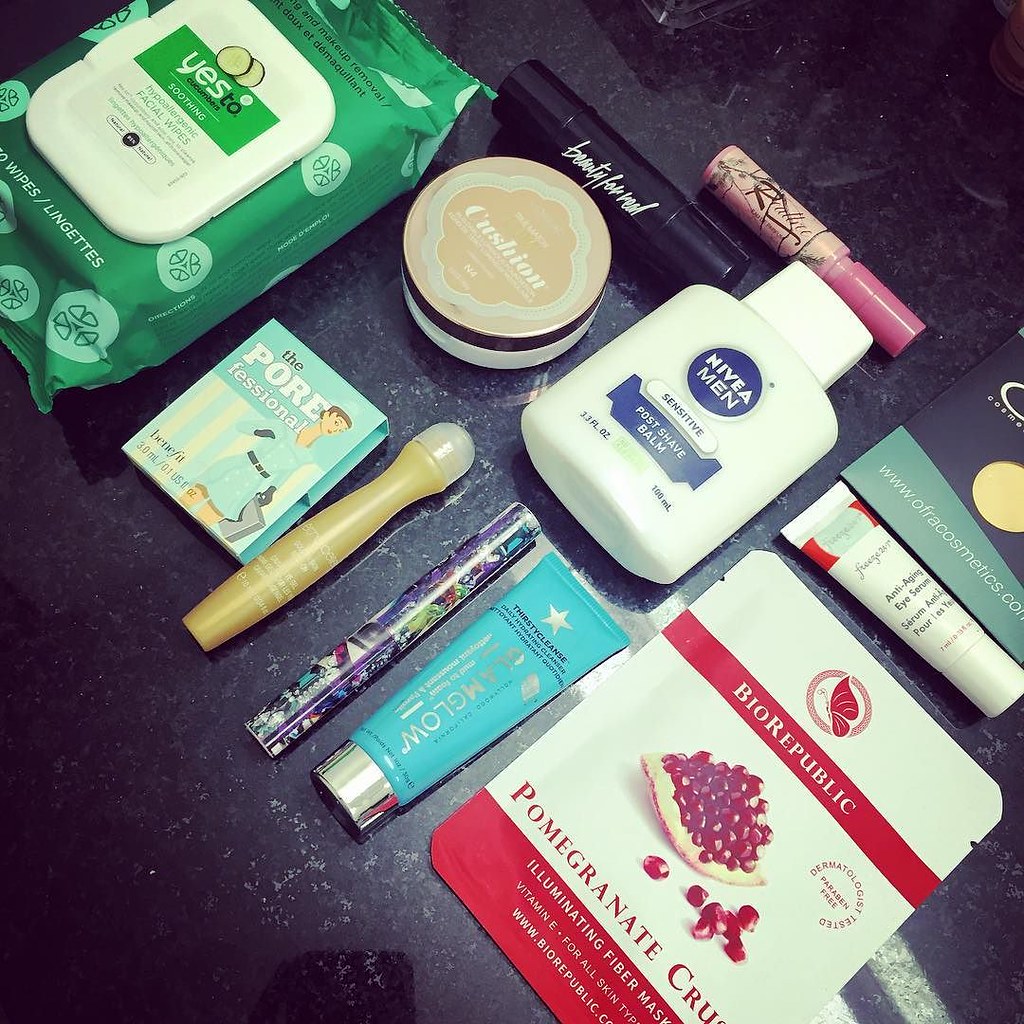A detailed collection of assorted personal care products is displayed. At the forefront, there is a box of cucumber-scented wipes, known for their refreshing and soothing properties. Next to it lies a compact cushion foundation, ideal for quick and easy touch-ups. Prominently featured is a bottle of Nivea for Men post-shave balm, designed to soothe and protect the skin after shaving.

Among the items, there are several tubes of products, including a green tube, though its exact purpose remains unclear, and a white tube with a red label. There is also a pink tube, which could either be a lipstick or a lip balm, adding a pop of color to the array. A yellow packet lies flat, which seems to be part of a multipurpose product packaging.

Additionally, the collection includes a packet labeled “Big Republic” that intriguingly contains pomegranate-scented crumbs, possibly exfoliating material. A product specifically designed for pore cleansing is present, alongside a stick that might be designed to assist with the exfoliation process. There is also a possible mascara stick and another blue tube, rounding out the diverse assortment of personal care items. This eclectic mix highlights a comprehensive approach to personal grooming and skincare.